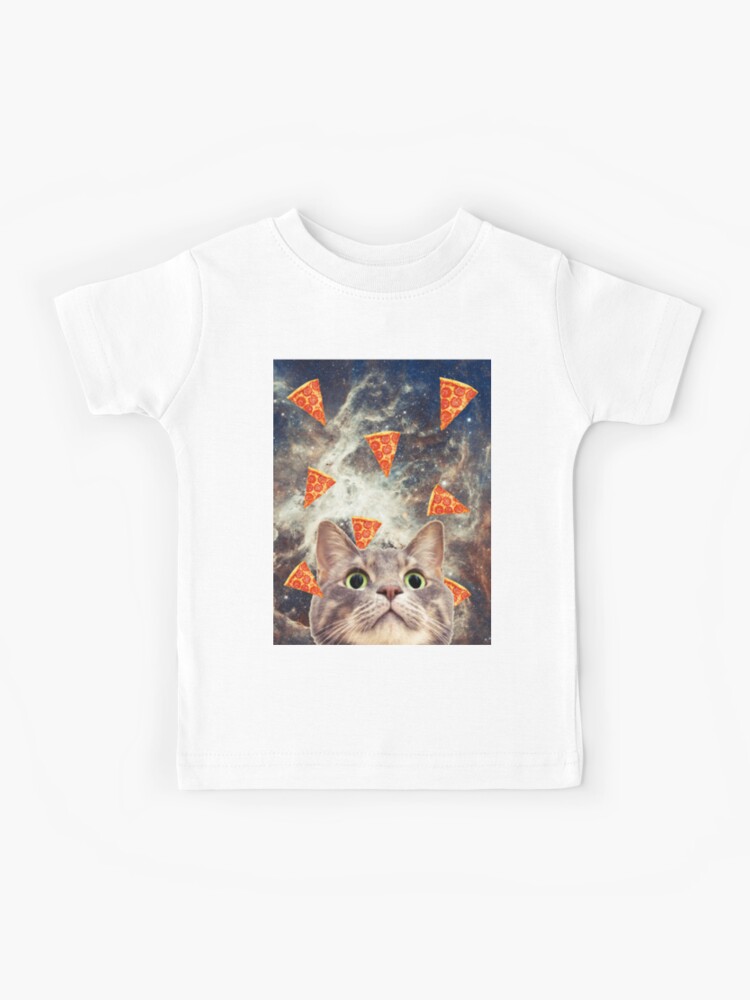This image showcases a plain white, short-sleeved, crew neck t-shirt featuring a printed rectangular design in the center. The design depicts a whimsical scene set in outer space, with a background of a deep blue starry sky. In the illustration, a gray tabby cat with tan and beige accents, highlighted by its cute red nose and light blue eyes, gazes upward in awe. Surrounding the cat, eight slices of plain pepperoni pizza are scattered, creating a playful, gravity-defying scenario. The cat's large, round eyes and look of intense curiosity add a humorous touch. This t-shirt appears to be a fun, lighthearted piece, possibly generated by AI, perfect for those who enjoy quirky, eye-catching designs.